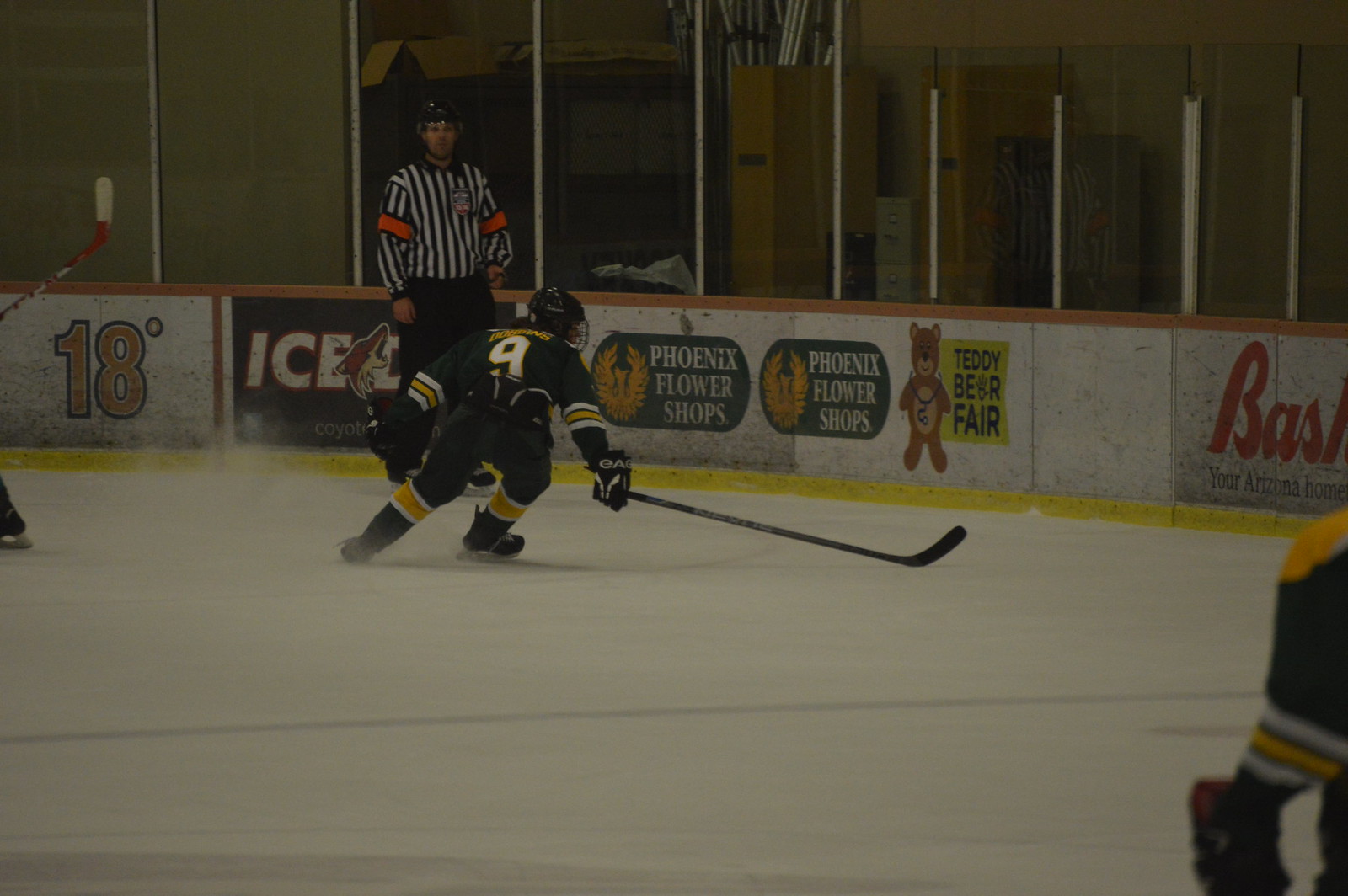In this photograph of a hockey game, the focus is on a player wearing the number nine jersey. The player is dressed in a black uniform with yellow stripes, including black pants, skates, gloves, helmet, and stick. He is lunging to the right, seemingly reaching for a puck, with his back toward us. To the left, a referee stands against the wall, watching the action unfold. The ice surface reaches about halfway up the image, bisected by a yellow bar along the bottom of the wall. Above the ice, the wall features several advertisements, such as "Phoenix Flower Shops" and "Teddy Bear Fair." The top of the image shows glass panels that separate the ice rink from the spectator area, though no spectators are present. Instead, behind the glass are some yellow cabinets and clutter, giving the impression that this might be a minor league game or a scene still under construction.